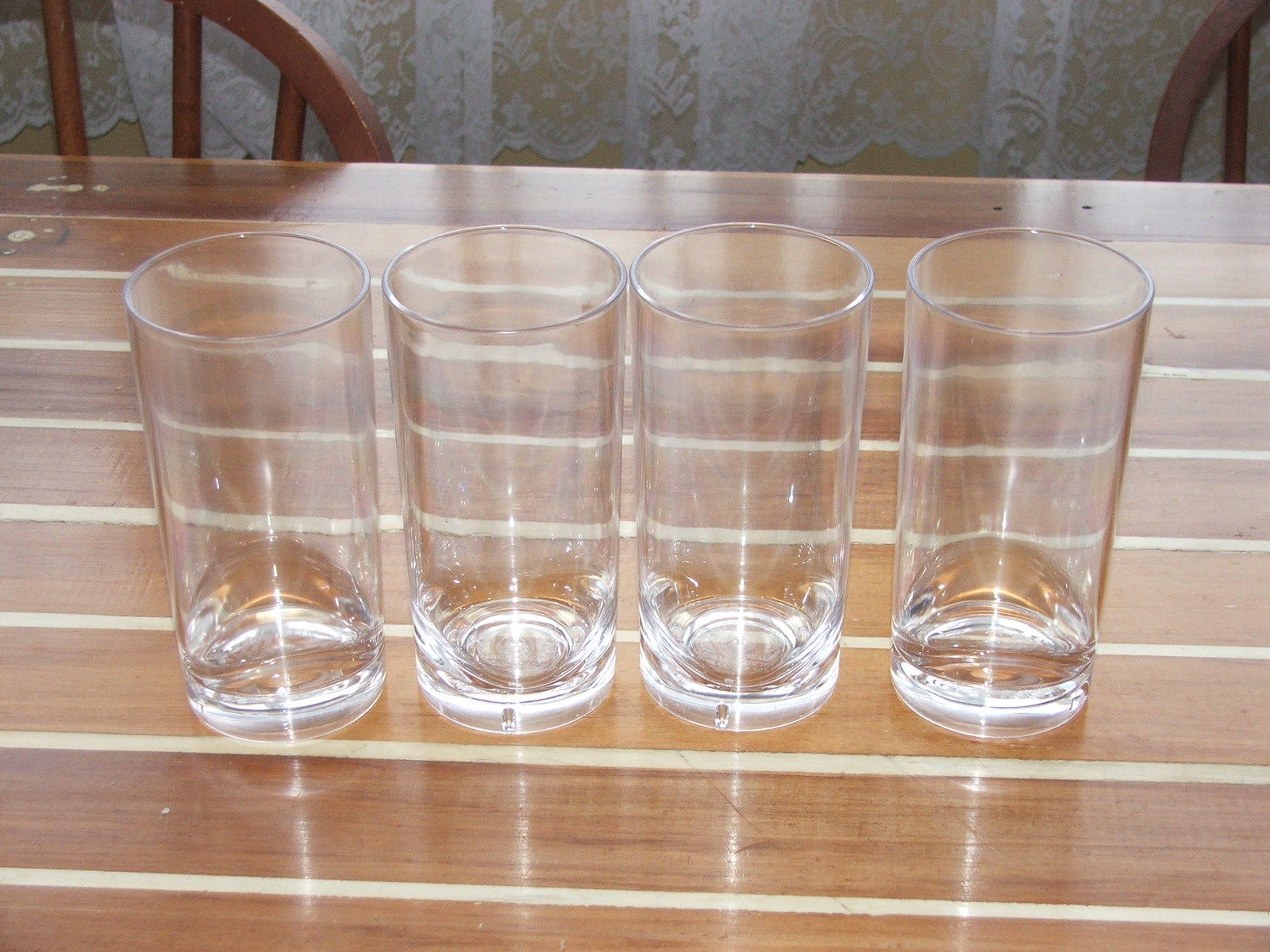The image depicts a wooden table made with slats of light and dark brown wood, featuring distinct white laminate lines. Centered on this table are four clear, clean, and shimmering glasses. The glasses are tall and narrow, with the two on the left and right differing slightly in shape at the bottom compared to the two in the middle. Behind the glasses, two wooden chairs with spindle backs are partially visible, characterized by their round and open-back designs. The chairs and table cast visible reflections due to light cascading through a window behind a white, semi-transparent lace curtain, adorned with floral embroidery. Beyond the curtain, patches of a golden-yellow painted wall can be seen. The ambiance suggests a neat and well-lit room.